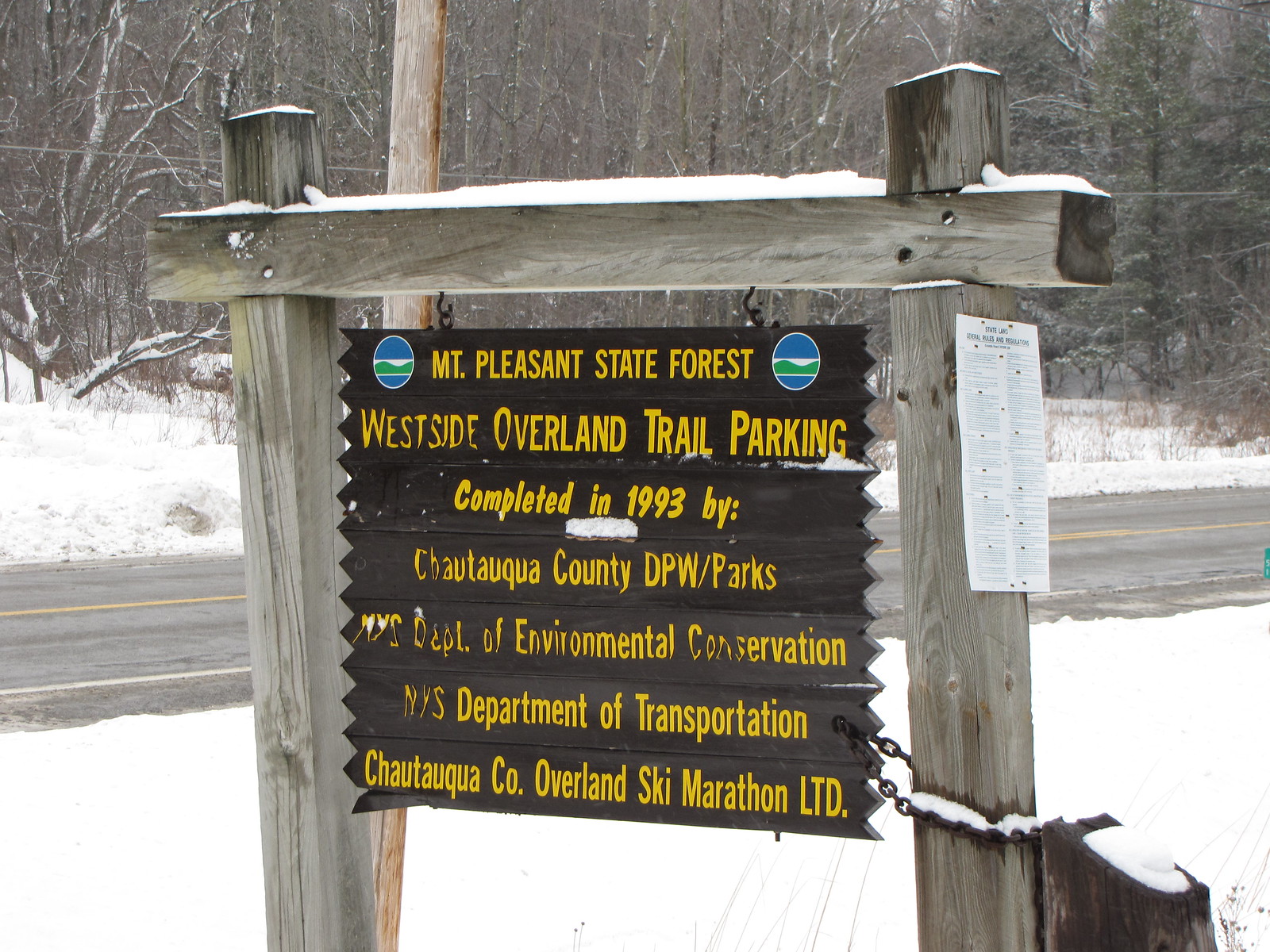In the photograph, a winter scene is depicted with a blanket of snow covering the ground and bare trees dusted with snow in the background. Dominating the foreground is a wooden fence in a grayish hue, adorned with a prominently displayed sign. The sign, encased in what appears to be a metal frame with silver edges, has a wooden aesthetic. It is primarily black with yellow text which reads: "Mount Pleasant State Forest. West Side Overland Trail Parking. Completed in 1993 by Chautauqua County DPW Parks, NYS Department of Environmental Conservation, NYS Department of Transportation, and Chautauqua County Overland Ski Marathon Limited." The sign also features a circular logo with blue at the top and bottom and a green swoosh symbolizing mountains. This informational sign marks the entrance to a park, nestled near a highway, setting a serene, wintry backdrop for visitors.